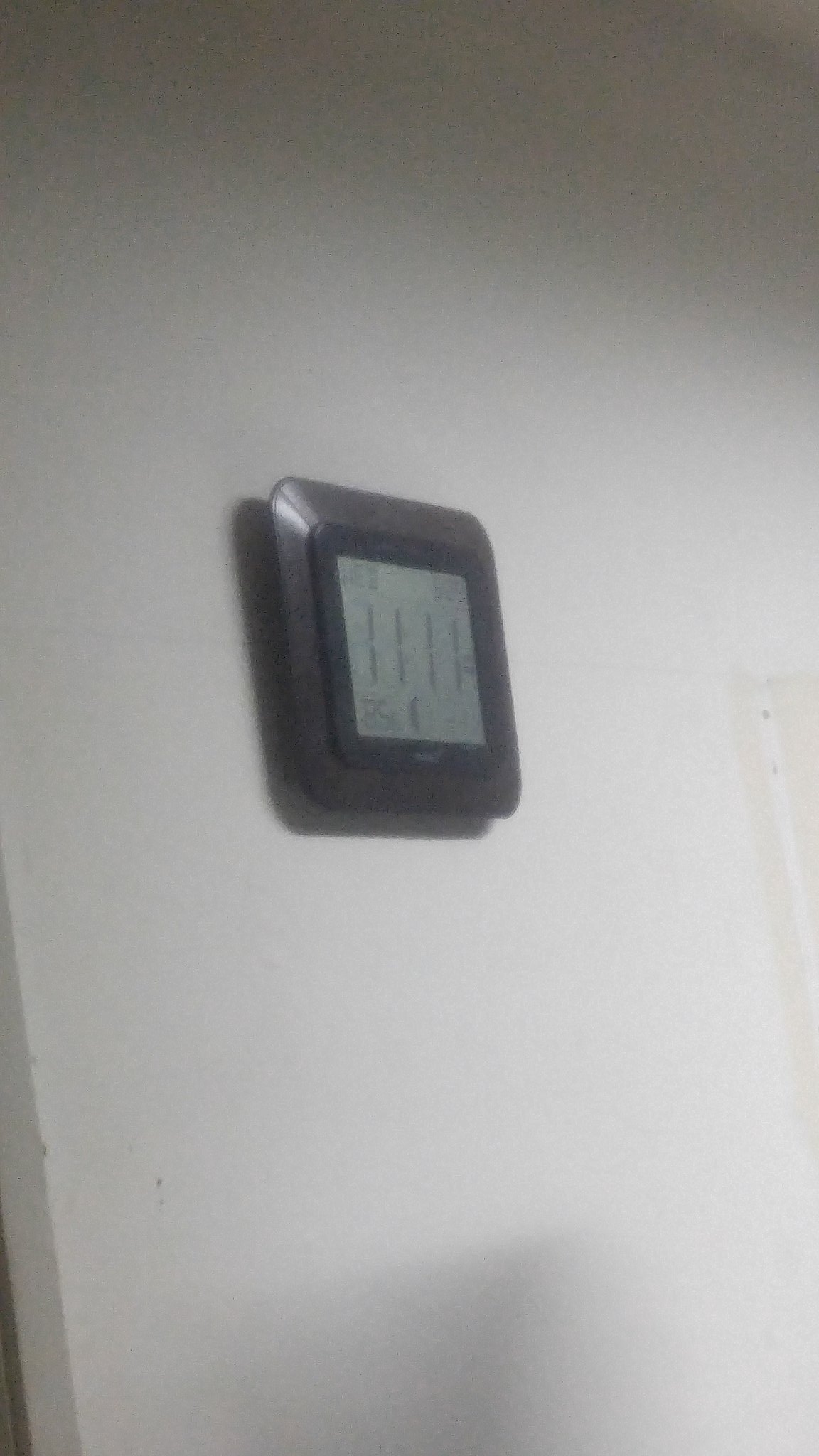The photograph captures a digital clock mounted on the center of a dull white wall, seen from a first-person perspective at a roughly 45-degree angle to the left. The clock, a stubby rectangle or square with rounded sides, boasts a sleek, reflective black frame likely made of plastic. This frame encloses a darker, inner border, also black but of a different material suggesting it might be more matte. The LCD screen, a grey rectangle within this frame, prominently displays the time "11:11". Additional details on the screen include partial numbers and symbols, one of which appears to indicate lunar phases with a half-moon icon, though specific elements are obscured due to the viewing angle. The slight shadow on the wall suggests either an unseen object or the photographer's presence, enhancing the image's depth.